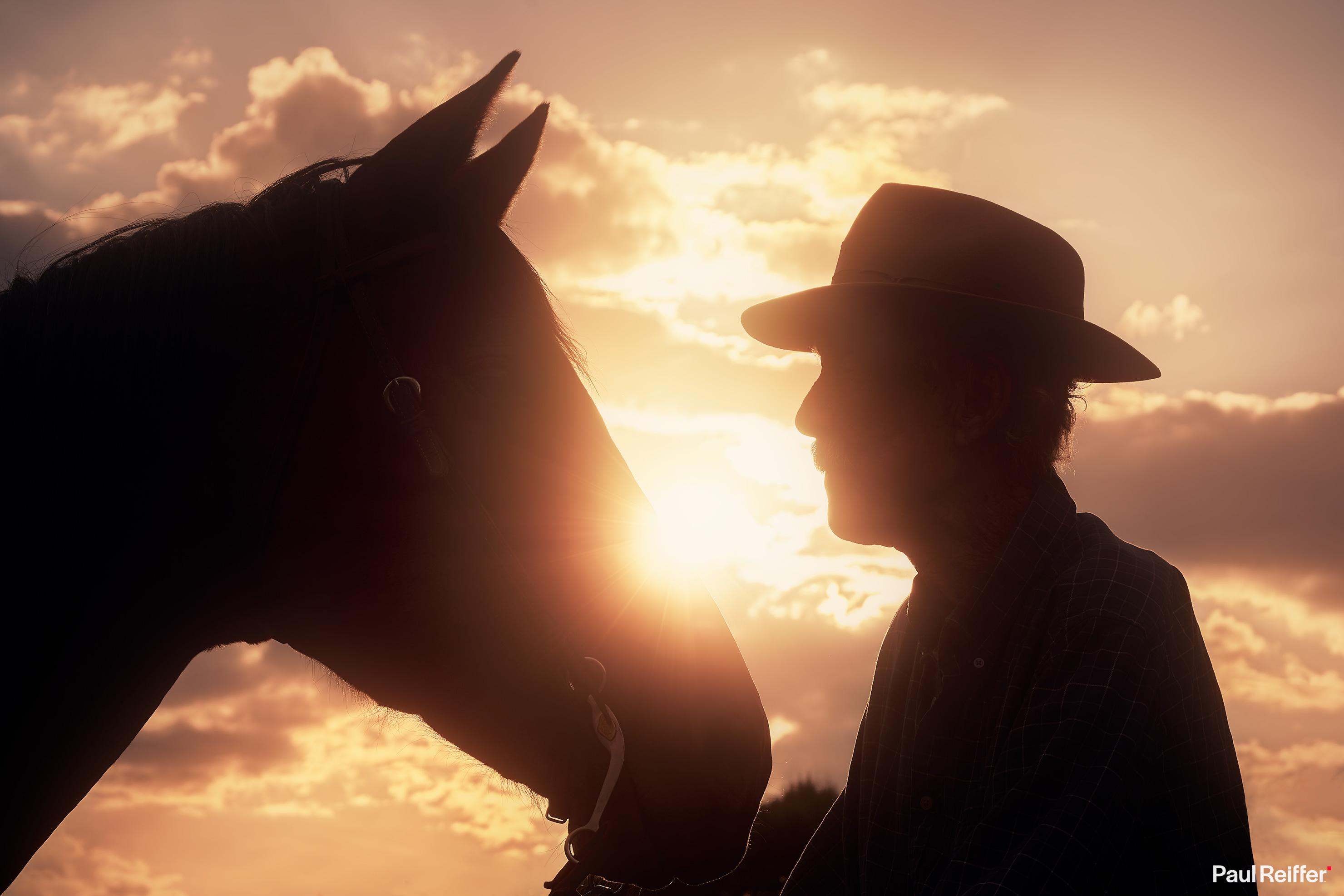In this artistic photograph, taken by Paul Reifer and credited at the bottom right, a close-up silhouette captures an intimate moment between a male figure and a horse. Set against an orange-tinted sky with the sun partially obscured by clouds, the image intensifies their shaded forms. The man, identifiable by his cowboy hat, stands on the right, facing and almost touching noses with the horse on the left. Only the head, neck, and part of the horse's body are visible, along with a contraption in the horse's mouth. The serene yet striking scene highlights their bond, framed by the ethereal glow of the setting sun at the center, casting them into a delicate silhouette.